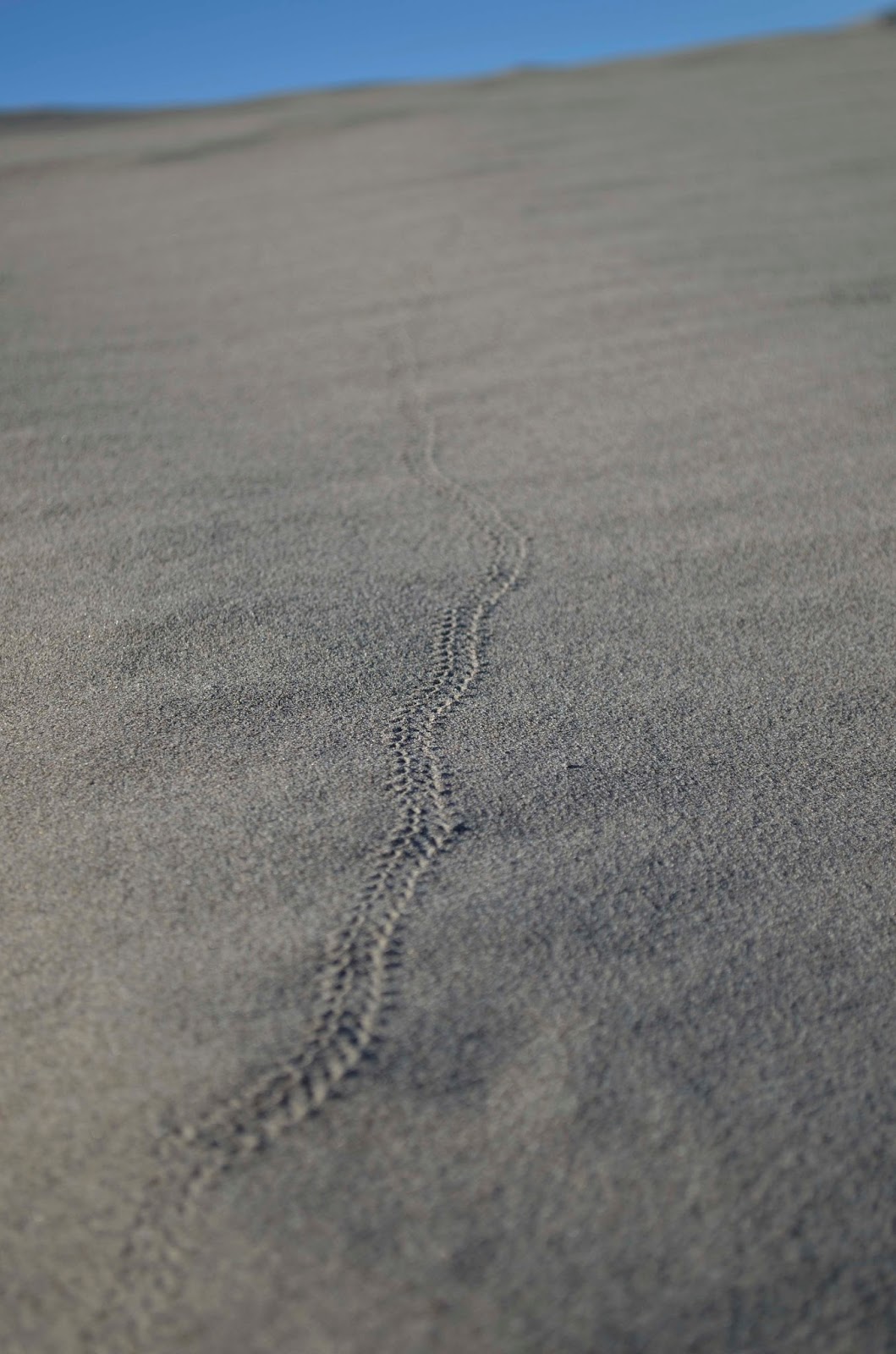In this image of a vast, open desert, the sandy, gritty ground stretches out under a clear blue sky that occupies the upper portion of the scene. Dominating the foreground is a single, winding track that weaves through the sand, coming from the bottom left and curving as it passes through the middle towards the distance. The track, about one to two inches wide, is distinctly defined and suggests the movement of something with a deep tread, possibly a snake or a deep-treaded tire. The sand is a grayish-brown hue, and the landscape appears mostly flat, though there are slight divots and hints of hills far off in the distance. The sky, bright and unblemished, adds a contrast to the otherwise monotonous sandy expanse.